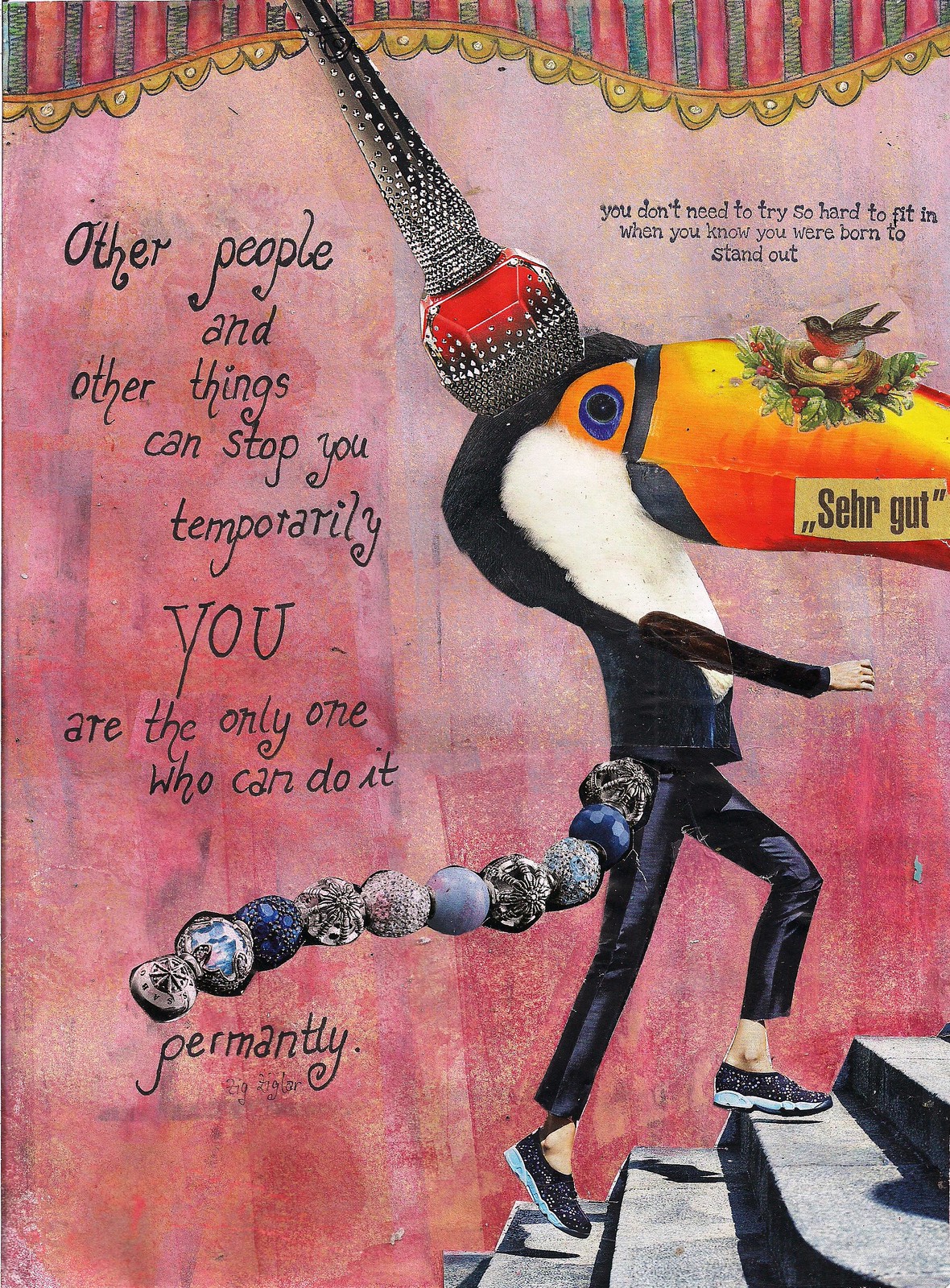The image is a detailed and vibrant poster that features the central figure of a human-animal hybrid walking up a gray cement staircase. The background is a grainy mix of red, rusty orange, and yellow hues, creating a warm yet dramatic setting. At the top of the image, a banner resembling an elaborate circus or cinema curtain drapes down with black and red stripes and gold trim.

The hybrid creature combines various elements: from its feet to its waist, it appears human, wearing black shoes and black leather pants that end just above the ankles, fully revealing its feet and ankles. The upper half of the body transitions into the head of a toucan bird, characterized by an orange, yellow, and black beak, blue eyes, and black and white fur. Notably, an upside-down microphone adorns the top of its head. Additionally, the creature has a tail composed of circular beads in various styles and colors, mainly blue, pink, and dark hues.

The poster features motivational text in black: on the left side, "Other people and other things can stop you temporarily; you are the only one who can do it permanently," and on the upper right side, "You don't need to try so hard to fit in when you know you were born to stand out." On the bird’s beak, enclosed in a light brown rectangle, is the text "Sir Gut."